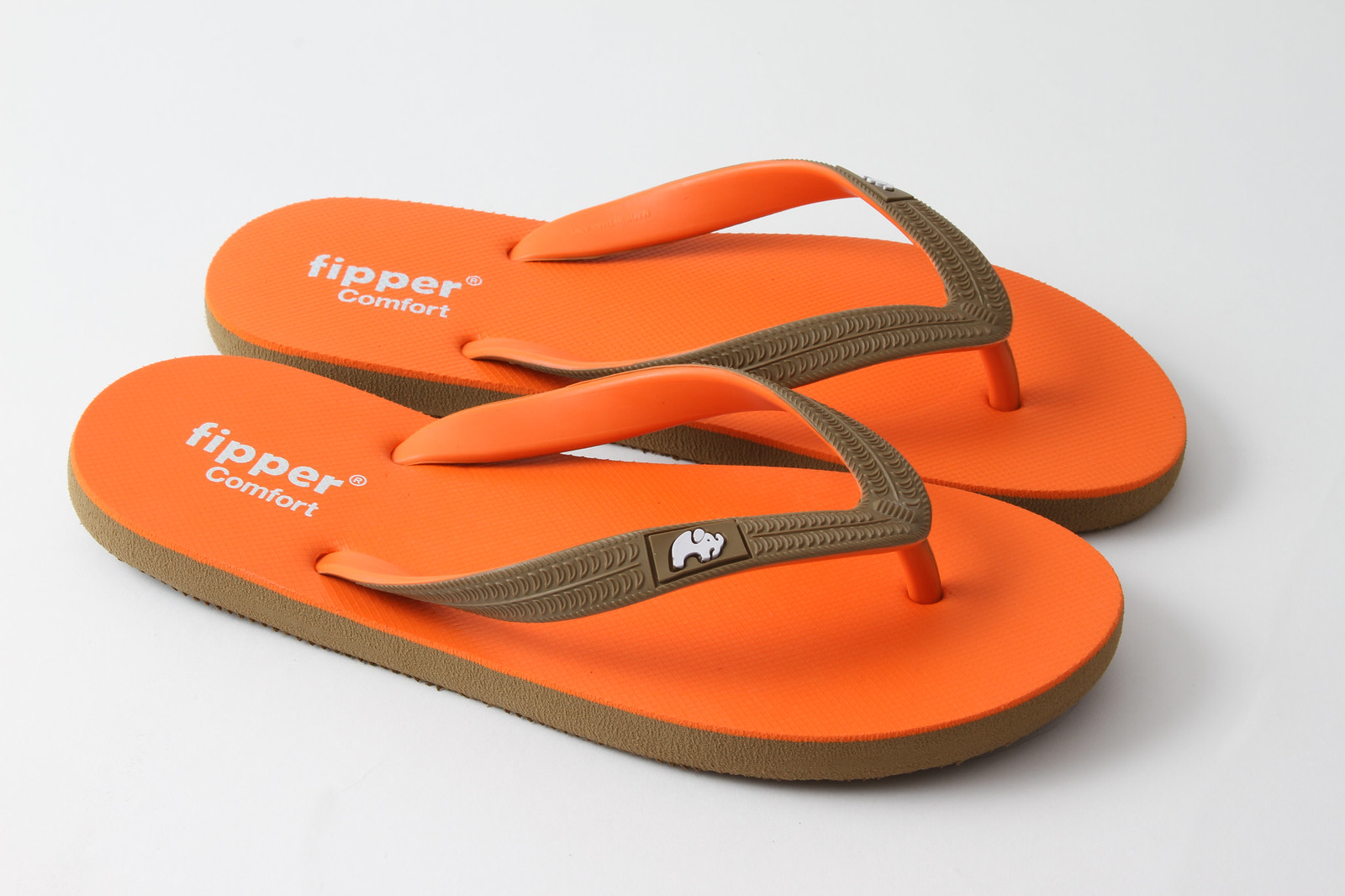This close-up professional photograph showcases a pair of flip-flops, known as thongs or sandals, prominently used in advertising, catalogs, and promotional materials. The flip-flops are primarily orange with distinctive brown straps and a brown edge around the bottom sole. A small, stylized white elephant logo is visible on the brown straps. The sandal soles feature the text "Fipper Comfort" in white, accompanied by a registered trademark symbol (®) next to 'Fipper'. Ensuring a clear view of the brand name and logo, the flip-flops are positioned side-by-side on a plain, light-colored background, with the toes facing the right-hand side of the image. This image appears meticulously crafted for product or business purposes.